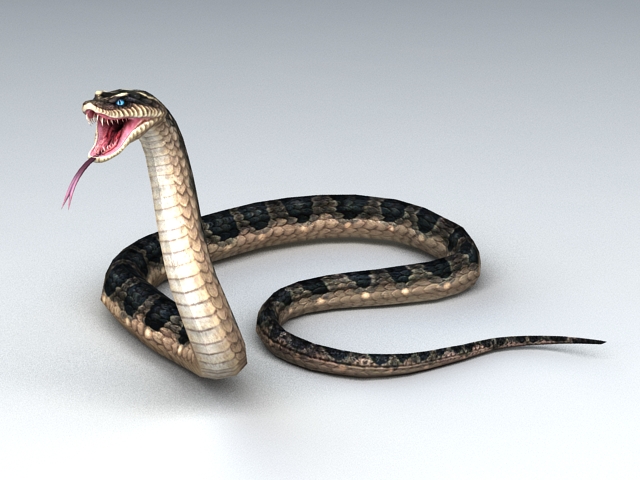This is a detailed, realistic digital illustration of a snake set against a gradient background that transitions from gray at the top to a lighter white color at the bottom. The snake, depicted in an aggressive, upright pose with its mouth open and tongue extended, showcases vibrant blue eyes and visible fangs. Its coloration features a dark green back with black stripes, while its underside presents varying shades of beige and white. Additionally, a slight white stripe can be seen across the back of its head. The snake's tail extends towards the right edge of the image, and the overall composition contains no text.